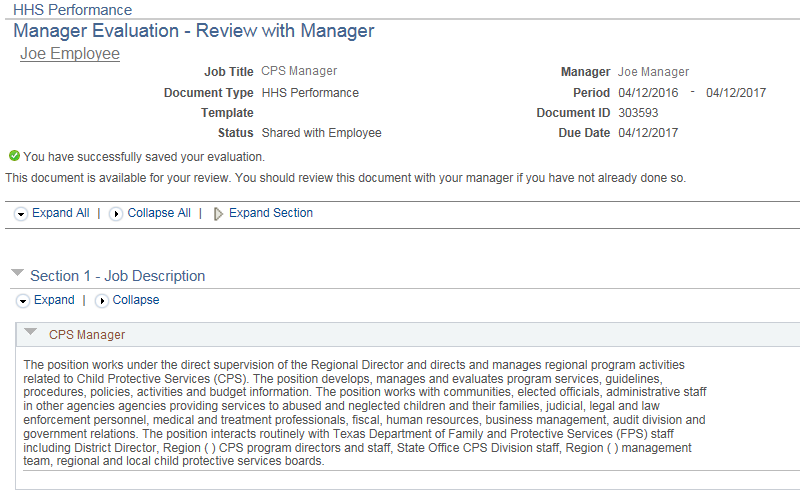The webpage is designed with a white background and primarily light gray text. In the top left corner, there is the acronym "HHS" in capital letters, followed by the word "performance." A thin gray line runs horizontally across the page beneath this heading.

The title "Manager Evaluation - Review with Manager" is prominently displayed in blue text. Below that, the name "Joe Employee" is underlined in gray text. To the right, detailed review information is listed, including:
- Job Title: CPS Manager
- Document Type: HHS Performance
- Template Status: Shared with Employee
- Manager: Joe Manager
- Period: 4-12-2016 to 4-12-2017
- Document ID: 303593
- Due Date: 4-12-2017

Beneath this information, there is a green verification checkmark alongside a confirmation message in text: "You have successfully saved your evaluation. This document is available for your review. You should review this document with your manager if you have not already done so."

Further down the page, there are options to "Expand All," "Collapse All," or "Expand a Section." Following these options, "Section 1: Job Description" is noted, with the ability to expand or collapse this section.

A light blue ribbon spans across the page with "CPS Manager" written in red text. Below this ribbon, a detailed paragraph describes the responsibilities and expectations of the CPS Manager position.